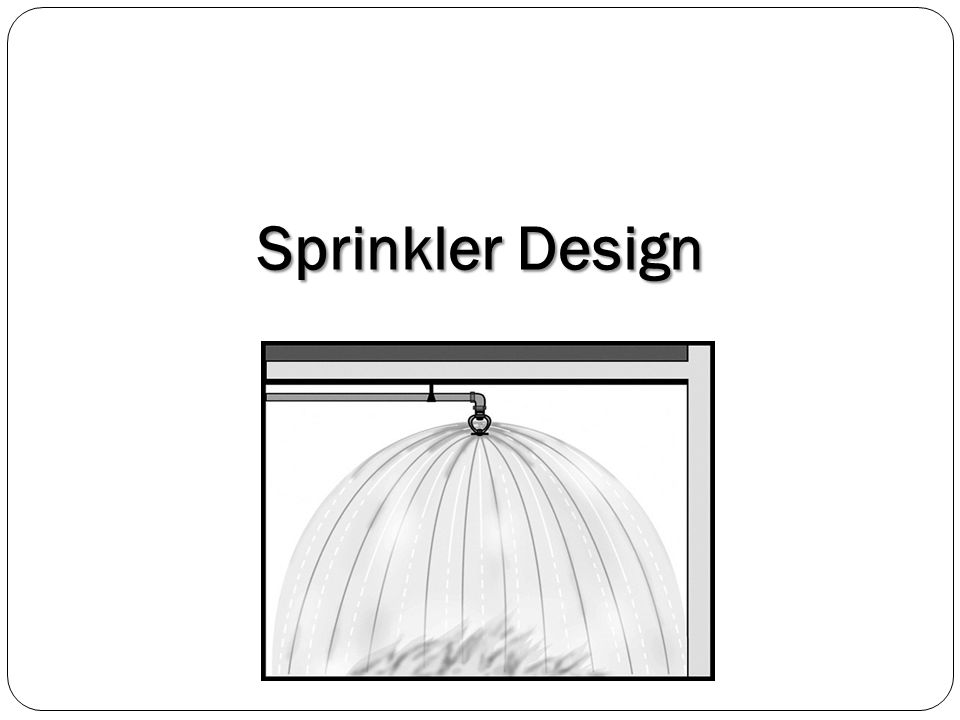The image depicts a black and white technical drawing in a landscape orientation, presented in an old-style educational slide format. The slide features a white background with a thin black border that has rounded edges. In the upper center of the image, bold black text reads "Sprinkler Design." Below this text, in the bottom center, is a framed illustration of a sprinkler system. The sprinkler is shown as a gray, dome-shaped nozzle connected to a metal pipe that comes from the top left and bends downward, dispersing water in a half-circle pattern resembling an umbrella. Thin lines represent the water spray, and there are small sketches of flames beneath the sprinkler, indicating its use in a fire suppression context. The entire composition, including the detailed technical drawing of the sprinkler system and the informative text, is rendered in varying shades of black and gray, creating a monochromatic, technical presentation style.